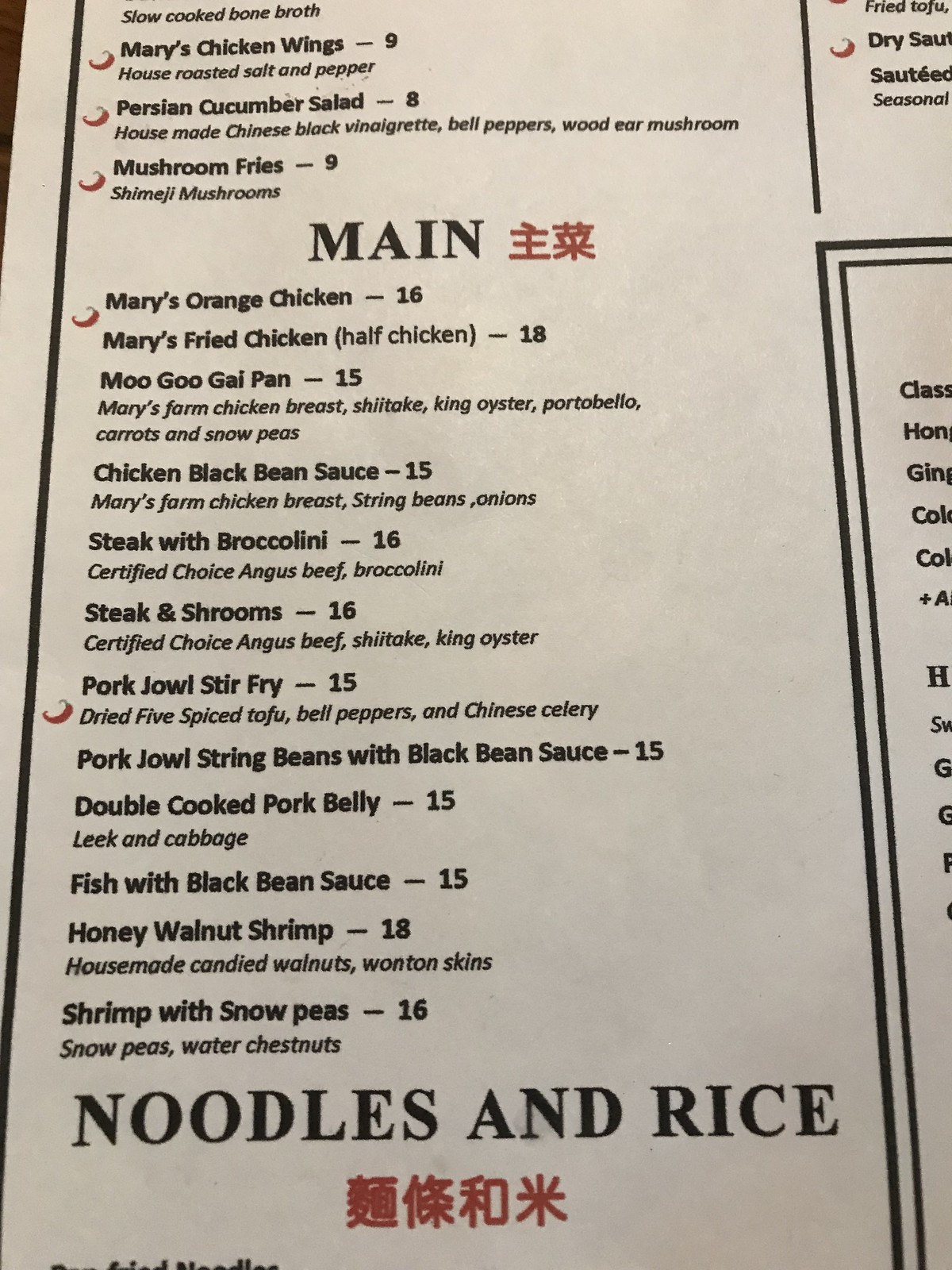This photograph captures the detailed design of a restaurant menu, likely from a Chinese establishment, presented on a white background with precise black and red detailing. The left edge of the menu is adorned with a thick black border, and another vertical black line runs parallel to the left border, demarcating a specific column of the menu. Just above a secondary black border, this line stops, suggesting a segmented structure for the menu layout.

The header of the menu prominently displays the word "Main" in a bold, Times New Roman-like uppercase font, complemented by a distinctive red Chinese or Japanese symbol beside it. Further down, the sections dedicated to "Noodles and Rice" feature four red Asian symbols, adding an authentic cultural touch.

Red chili icons are strategically positioned next to certain dishes to signify spice levels, with five such indicators visible in the main column and one more in the top right corner, likely serving as a caution for diners about the spiciness of some items. Each dish listed includes both a description of the ingredients and the price.

The primary focus of the photograph is on the "Mains" section, but it also partially captures additional details from the right-hand side of the menu. This section appears to be within its own bordered block, maintaining consistent use of lines for a neat, organized structure.